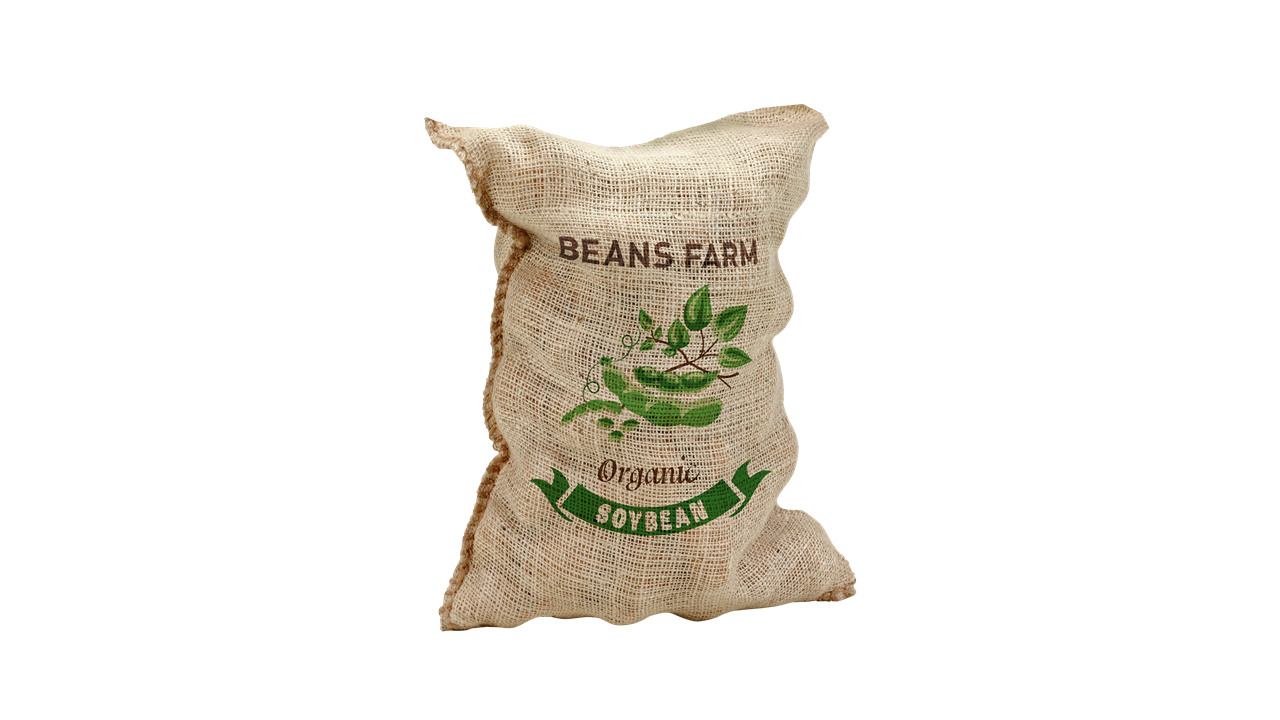The image depicts a vertically oriented, natural burlap bag set against a clear, white background. At the top of the bag, the words "BEANS FARM" are prominently displayed in brown capital letters. Centrally featured is a detailed graphic illustration of green soybean pods attached to a green stem with leaves, accompanied by smaller disconnected soybeans and a subtle green swirly design. Below this illustration, the word "ORGANIC" is elegantly scripted in brown cursive. At the very bottom of the bag, a green ribbon banner bears the word "SOYBEAN," with the letters in the natural burlap color of the bag itself. The overall presentation is rustic and farm-themed, highlighting the organic nature of the product.